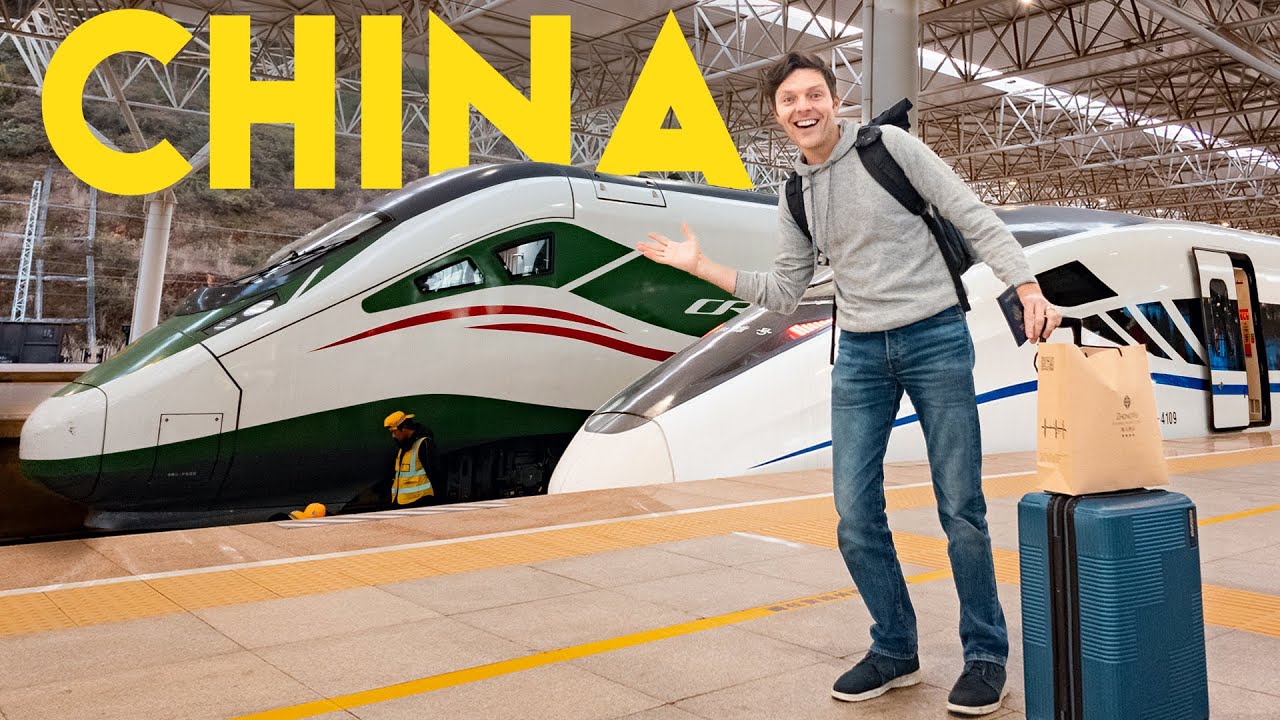In a bustling high-speed train station in China, a cheerful Caucasian traveler, likely a YouTuber, stands prominently in the foreground, smiling broadly. He is dressed in a gray hoodie with dangling drawstrings, blue jeans, and dark sneakers. A black backpack is slung over his shoulders, and he grips a blue hard-shell suitcase adorned with a brown shopping bag on top. His right arm is outstretched, pointing towards large, bright yellow capital letters reading "CHINA" in the top left corner of the image. Behind him, two sleek bullet trains—one white with green and red accents and the other white with navy blue markings—are stationed on tiled platforms. The station's metallic, grid-like ceiling looms above. Two men in high-visibility vests work on the tracks near the trains, giving the impression of a dynamic and modern travel hub.